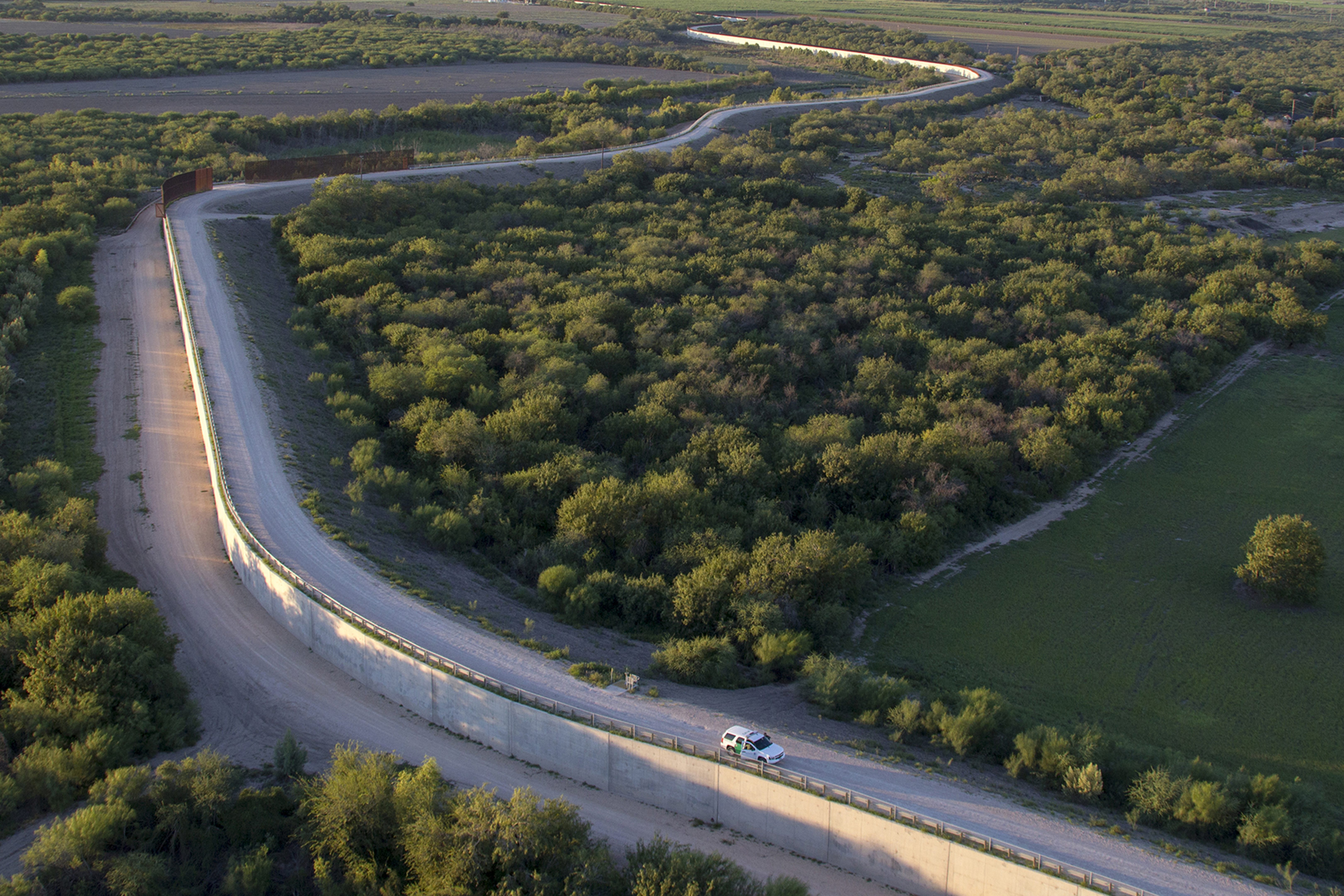This image captures an aerial view of a winding highway snaking through a vast, lush forest landscape. The road, which appears elevated due to a visible concrete barrier along its edge, meanders from the bottom left of the image to the center top. A lone white SUV is visible near the bottom of the picture, emphasizing the emptiness and tranquility of the scene. Surrounding the highway, the dense green forest is contrasted by a small patch of open grassland at the bottom right. The overall scene is vividly colored, with the bright greens of the forest and the neutral gray of the road standing out under what appears to be a sunny sky. There are no people, houses, or additional vehicles in sight, highlighting the secluded and serene nature of this outdoor setting.